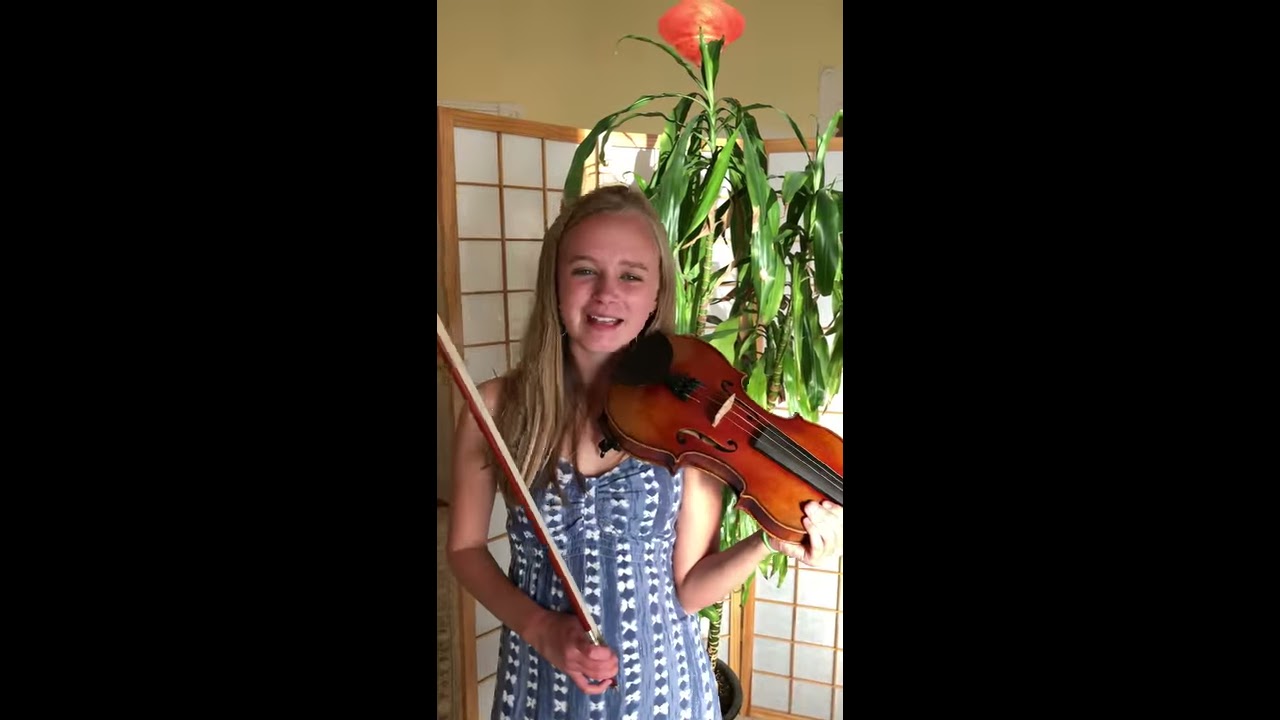This detailed photograph features a young girl standing centrally in a room, smiling for the camera as she holds a violin in her left hand and a bow in her right hand. She wears a blue and white dress. The room behind her has light yellow painted walls and a white and brown rice paper room divider. Adding a touch of greenery, a tall tropical indoor plant, approximately five to six feet in height with green leaves and a red flower on top, is positioned behind her in a pot. The photograph is bordered with two-inch wide black vertical panels on either side, measuring roughly seven inches wide by five inches tall. The image lacks any text or additional graphics, merely showcasing a high-quality photograph of the girl with the violin, framed by black borders. Hanging in the room, adding a pop of color, is a red pendant light fixture.